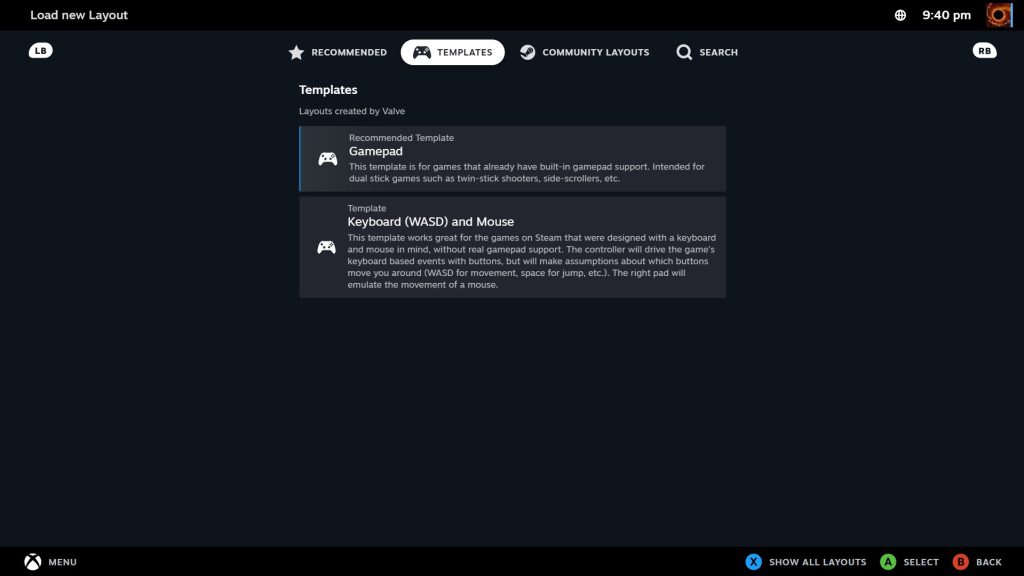A screenshot of an Xbox-related interface, most likely a website, app, or window. The top section of the screen displays "Load New Layout" with a menu bar on the left and a clock showing "9:40 PM" on the right. The background of the interface is predominantly black.

The main content area features several sections with white text, making navigation intuitive. At the top, prominently highlighted, is "Recommended Templates," followed by "Community Layouts" and a "Search" option. Below these headers, two highlighted templates are displayed with detailed descriptions.

1. The first template, titled "Gamepad Recommended Template," is designed for games with built-in gamepad support, ideal for dual-stick games such as twin-stick shooters and side-scrollers.
2. The second template is "Keyboard (WASD) and Mouse." This layout is suitable for games on Steam that are meant to be played with a keyboard and mouse, but with gamepad compatibility. Here, the gamepad buttons replicate keyboard actions, such as WASD for movement and space for jumping, while the right pad emulates mouse movements.

At the bottom of the screen, a horizontal menu bar is visible. On the left side of this bar, there's an Xbox icon labeled "Menu." On the right side, you'll find icons and text for various controls: a small "X" icon for "Show All Layouts," an "A" icon labeled "Select," and a "B" icon labeled "Back."

The overall design emphasizes usability and accessibility with clear, white text against a black background, effectively guiding the user through various customizable options for their gaming experience.